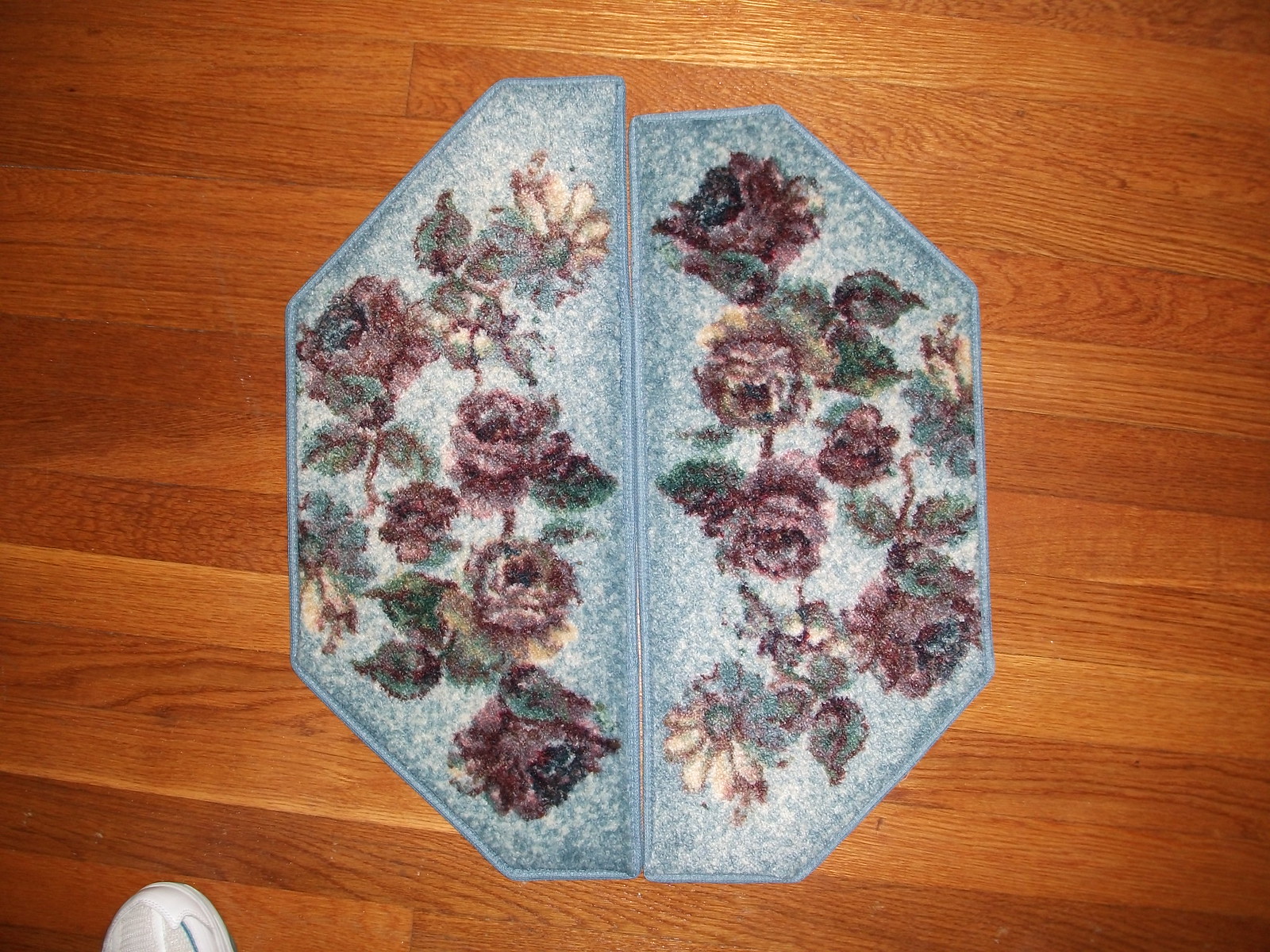This image showcases two intricately designed rugs placed on a brown wooden floor. The rugs are essentially identical in pattern and color, featuring a rich blue background adorned with flowers in shades of purple, maroon, red, and white, interspersed with green leaves. Despite the rugs being nearly the same, one is slightly taller than the other. The left rug, taller than the right, causes a slight misalignment when the two are placed together. Both rugs converge at their flat ends and then extend outward, forming a six-sided, slightly octagonal shape. On the left-hand bottom corner of the image, a glimpse of a white shoe with a blue stripe is visible, adding a subtle human element to the composition. The rugs' alternating lighter and darker blue hues accentuate the floral designs, making them stand out against the wooden floor.